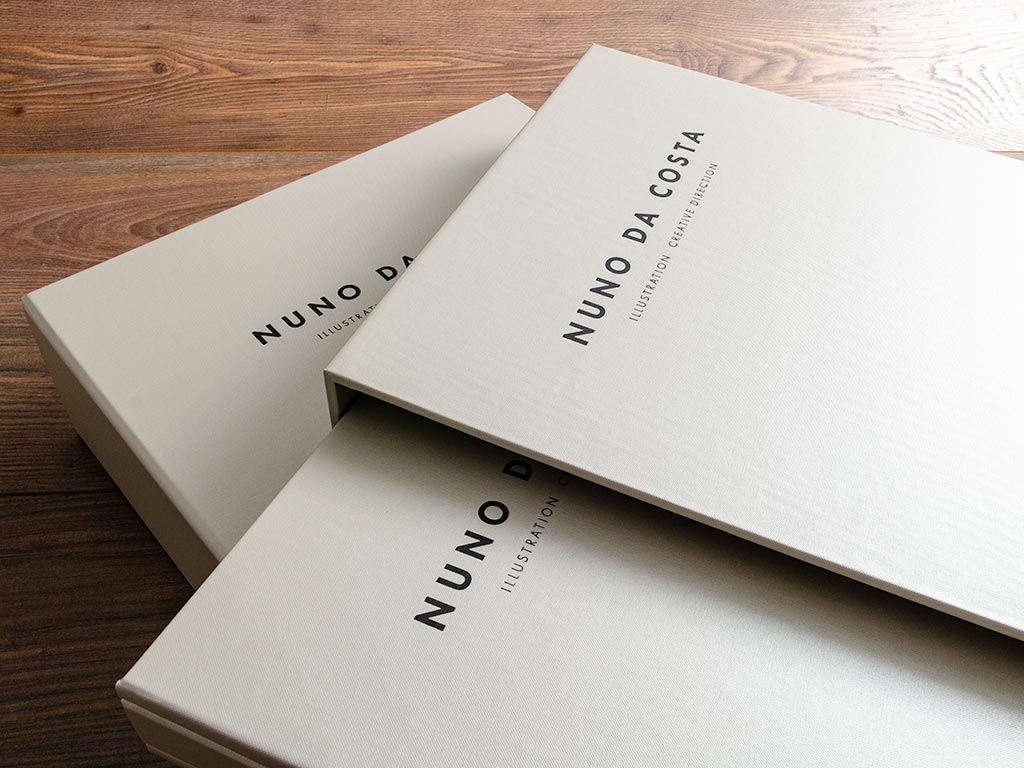The image shows three rectangular objects, which appear to be books or book cases, resting on a medium-dark brown wooden surface. The three objects share the same white top cover, inscribed with the black text "Nuno da Costa, Illustration, Creative Direction." This text is partly obscured on two of the objects but fully visible on one. The first object in the stack is being partially pulled out of its box cover, which is light cream in color with the same title printed on it. The second object is slightly visible and pulled towards the left corner of the photo, also carrying the same title in black, all-uppercase letters. The interiors of the objects seem different; one might be hollow, possibly serving as a case for the other two, but this is not entirely clear from the image. The detailed arrangement and similarities suggest a cohesive collection or series by the same author, Nuno da Costa.